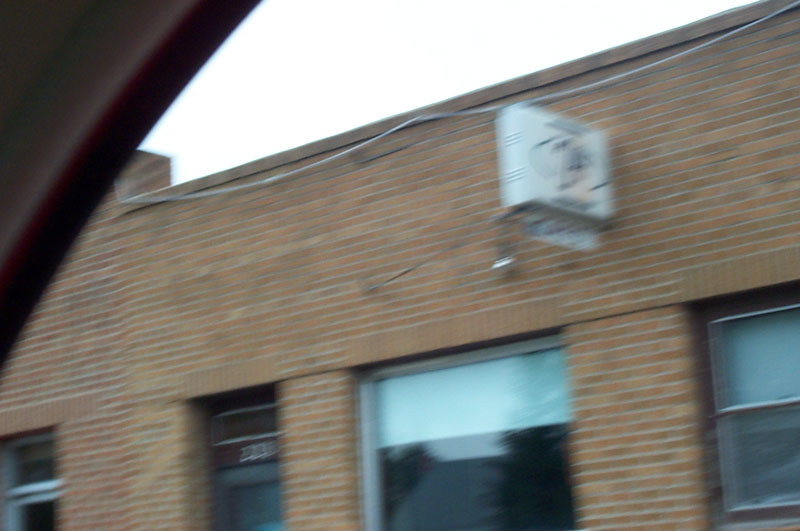This image depicts a very blurry scene of the side of a brick building, captured through the passenger-side window of a car, evident by the visible window frame in the upper left corner. The building's bricks are of a dark reddish-orange or maroon color. Two windows are visible, along with a door that appears to have an address number, which seems to read '283' though the blurriness makes it difficult to confirm. The door is on the first story, and there are multiple windows along this level, with one being notably slim and tall, possibly mistaken for another door. Additionally, a small white square sign with some sort of logo or lettering is mounted higher up on the building's exterior. The scene is set under a cloudy, murky sky, indicating the time of day to be during the day but with overcast weather.